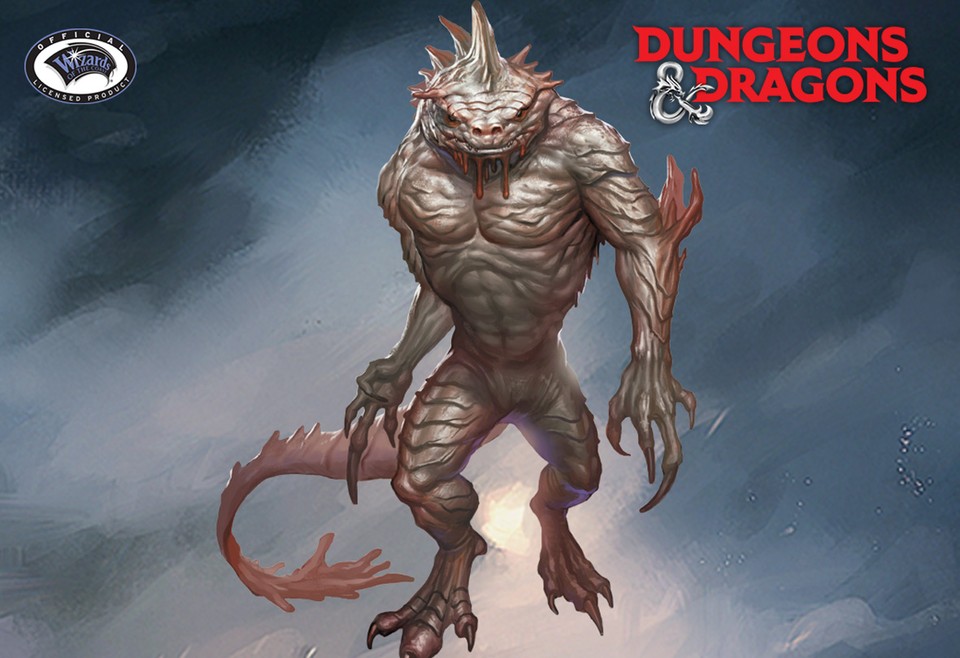The image showcases a muscular, bipedal creature from Dungeons and Dragons, with a prominent lizard or possibly snake-like appearance. This creature has no discernible neck and features spines that begin at its head and extend down its back, possibly reaching its tail. The body is predominantly light brown with pinkish tints around the spines on its shoulders and tail. The creature appears to be drooling blood from its mouth, adding to its menacing appearance.

The background of the image is a gray and black watercolor, reminiscent of a cloudy, somber sky. Displayed in the top right corner is the Dungeons and Dragons logo in red capitalized font, with an ampersand styled like a worm or dragon breathing fire. The top left corner features the official Wizards of the Coast seal, indicating the image is an official licensed product.